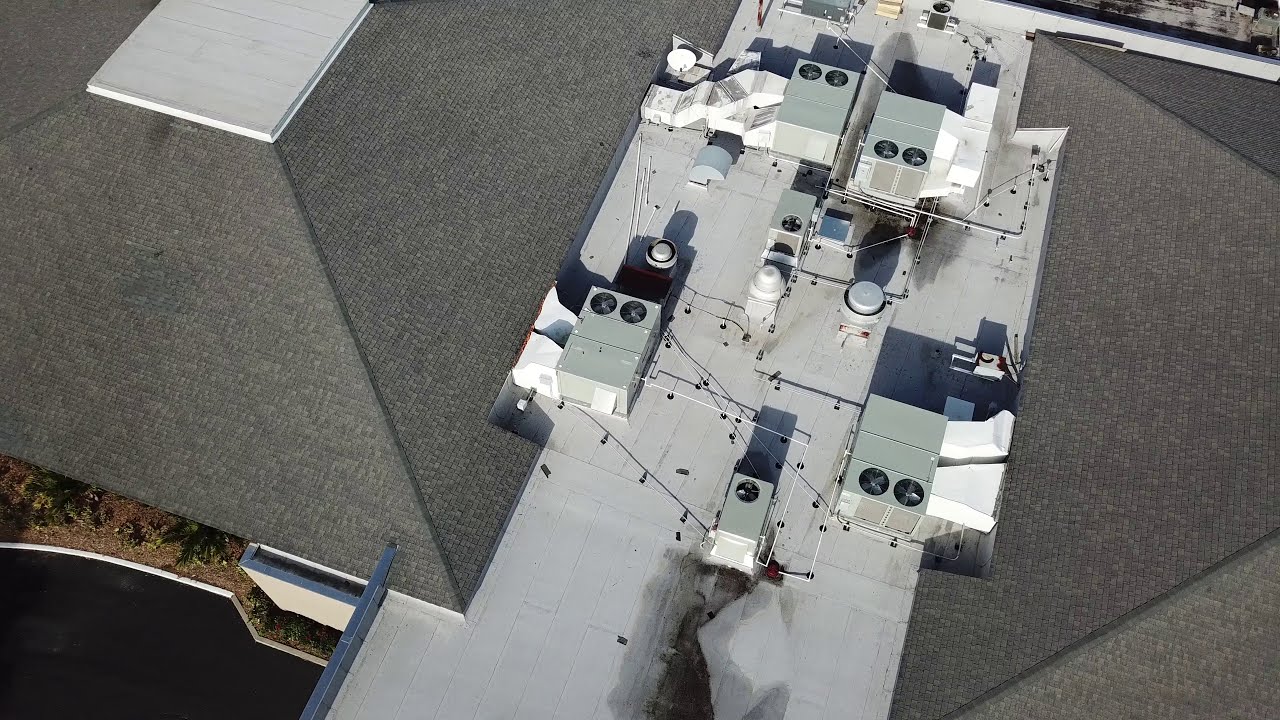The photograph is an overhead view of a large building's roof during daytime, bathed in natural light. The roof features a combination of a flat central portion and pitched sides covered with dark gray shingles. Prominently, the flat section is populated with numerous metal components including at least four or five rectangular silver boxes connected with pipes, likely air conditioning units or other cooling and refrigeration machinery. Additionally, silver cylinders and white air ducts are scattered across the gray paneled surface. The image also reveals parts of the building's architecture, with two pyramid-shaped, angled roofs flanking the flat portion and some visible shrubbery and landscaped plants encircling the building. There is a black tarmac road in front of the structure and a hint of grass in the bottom left-hand corner, providing a full, clear view without any text or numbers.